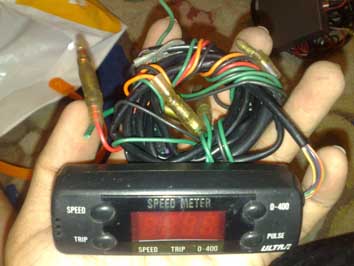A detailed close-up color photograph shows a person's left hand, palm up, holding a small black electronic device labeled "Speed Meter." The device, which has a rectangular shape, is equipped with a digital display screen that appears to reflect red light, suggesting an LED display, although the device is currently unplugged. On the left side of the Speed Meter, there are two clearly labeled buttons, "Speed" and "Trip." On the right side, two buttons are partially visible; the top one is unreadable, while the bottom one mentions "Activate."

Nestled alongside the Speed Meter is a tangle of wires resting in the person’s palm. The wiring includes a large black wire accompanied by smaller green, orange, red, and yellow wires, some of which are covered with insulating sleeves while others are exposed. 

In the backdrop of the image, the floor is visible, possibly illustrating a plastic shopping bag in the upper-left corner and an indistinct square object in the upper-right. The setting suggests a casual environment, possibly a workspace or a home setting.